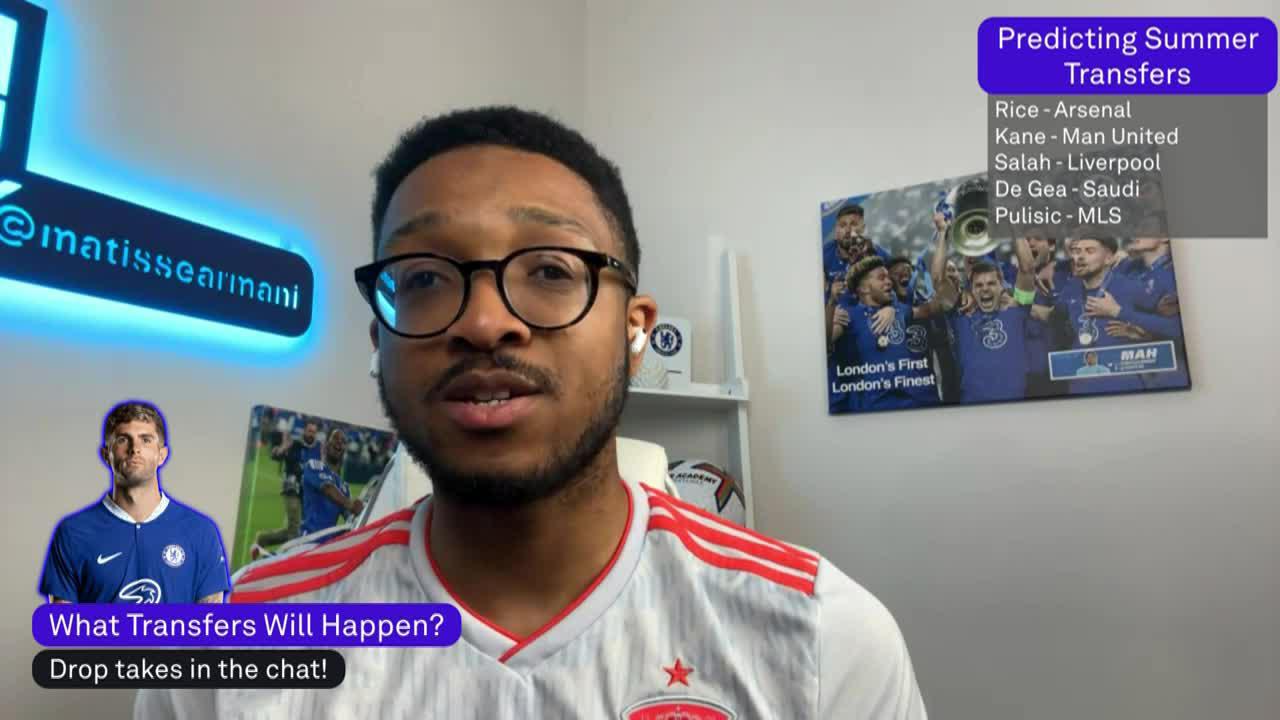A young man, possibly a college student, is depicted in this image, seated in a room that exudes a blend of casual comfort and fervent soccer enthusiasm. The room, likely a dormitory or personal bedroom, has walls painted a soft, creamy white, providing a neutral backdrop for various decorative elements. Prominently displayed on the wall is a vibrant soccer poster, capturing the dynamic spirit of the sport.

In the upper right-hand corner of the room, a digital or handwritten sign bears predictions for summer soccer transfers, listing notable players: Rice to Arsenal, Kane to Manchester United, Salah remaining at Liverpool, DiGiulia to Saudi Arabia, and Pulisic to Major League Soccer (MLS). The sign's bold headline reads, "Predicting Summer Transfers," while a blue subheading questions, "What Transfers Will Happen?" A contrasting black box at the bottom invites interaction with the prompt, "Drop Takes in the Chat."

Adding to the room's unique character, a lamp designed to project text onto the wall casts the phrase "Matisse Arnelli," which could be a personalized message or email address artistically crafted into the fixture. The overall scene is illuminated by the warm glow of this innovative lamp, casting intriguing shadows that enhance the room's inviting atmosphere.